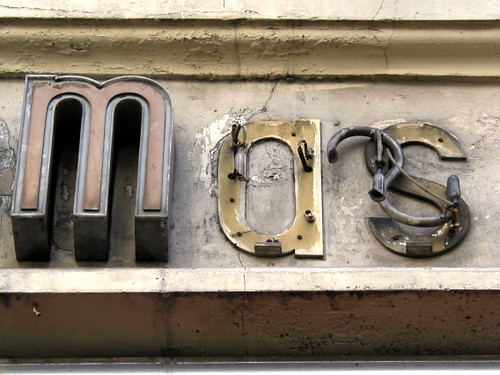In this close-up, full-color image, a possibly broken neon sign is captured in striking detail. The sign features the letters "M", "A", and "S." The "M" remains intact, illuminated in a vibrant red against its plastic casing, highlighting the typical effect of neon or argon gas lighting. However, the "A" and "S" are visibly damaged. The glowing outer plastic is missing, exposing a rusted, gold-colored metal plate that likely housed LED or neon elements. The backdrop appears to be a rooftop, with the sign situated on what seems to be a stone structure, though the perspective makes it challenging to identify the building's full exterior. The photograph emphasizes the contrast between the functioning segment and the deteriorated parts, offering a glimpse into the wear and tear of urban signage.